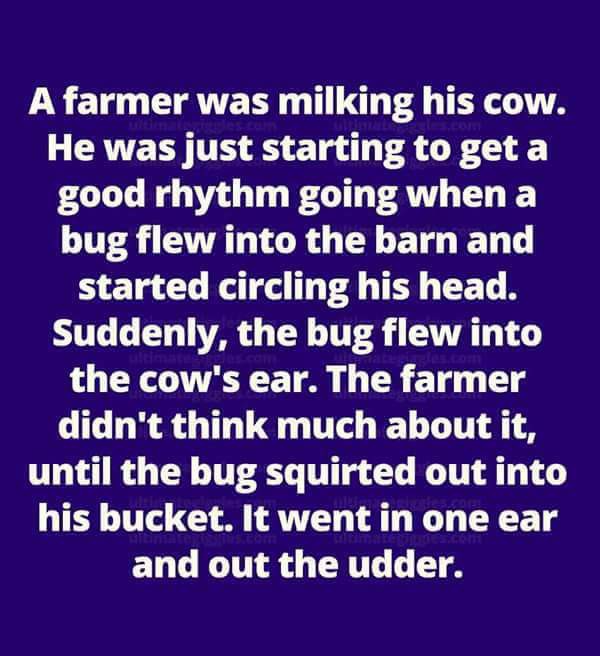The image is a meme or joke card often seen on social media platforms like Pinterest or Facebook. It features a simple design with a solid dark blue, almost navy purple background, and white text. The joke printed on the card reads: "A farmer was milking his cow. He was just starting to get a good rhythm going when a bug flew into the barn and started circling his head. Suddenly, the bug flew into the cow's ear. The farmer didn't think much about it until the bug squirted out into his bucket. It went in one ear and out the other." This phrase is a pun, playing on the idiom "in one ear and out the other," with "udder" humorously substituting for "other." The card is designed to resemble the type created for easy sharing online, emphasizing the text's humorous intent.